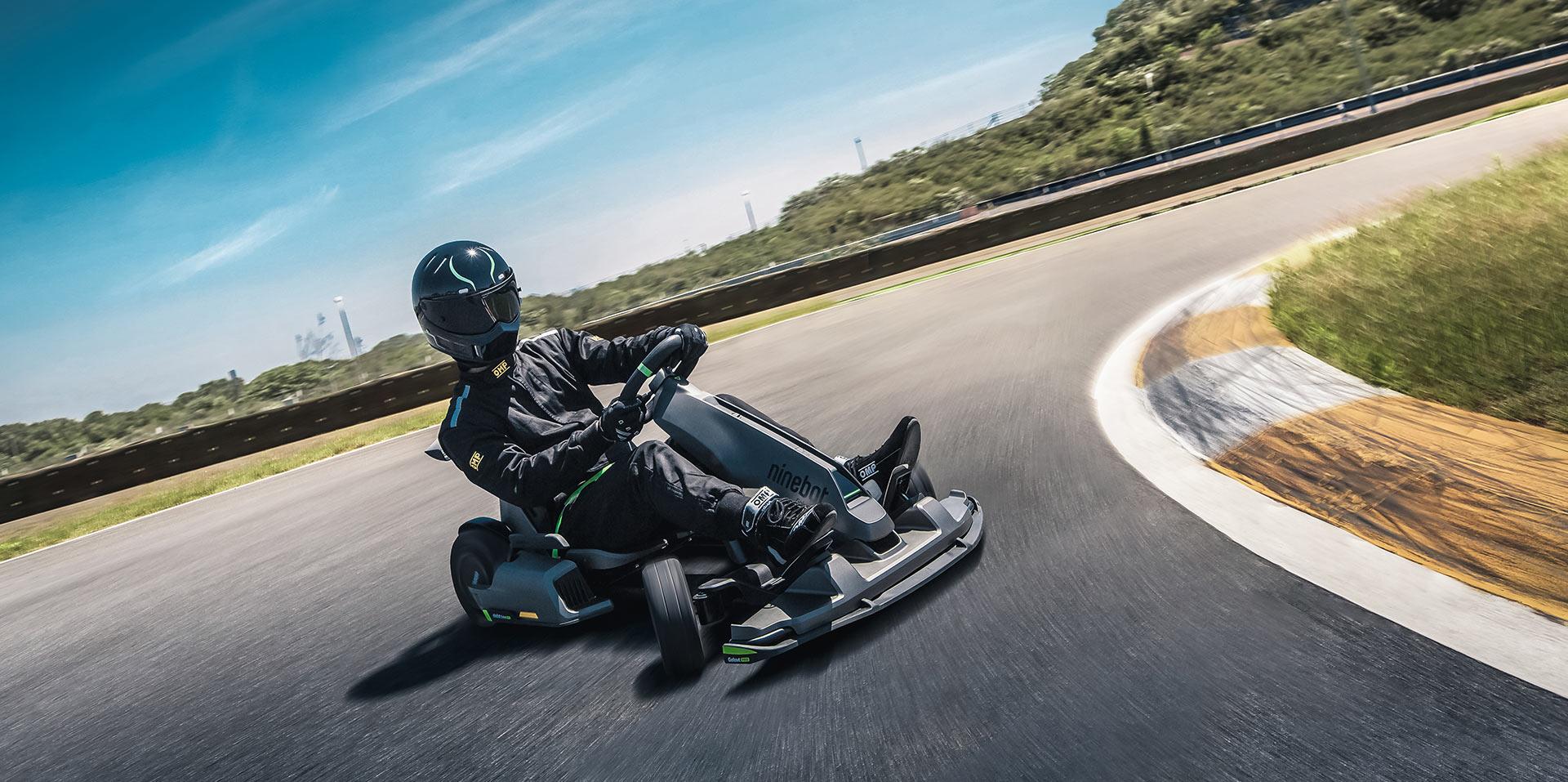In this outdoor photograph, a man is skillfully negotiating a turn on a go-kart racing track. The man, deeply engaged in his drive, is dressed entirely in black—black helmet adorned with light blue horn designs on the sides, a black jacket with blue light patterns and a yellow logo on his arm, black pants, black gloves, and matching black shoes with white stripes. The go-kart itself is gray and marked with the word "Ninebot" below its steering wheel, hinting at its electric nature due to the absence of a visible engine.

As he maneuvers through the turn, the back wheels of the go-kart slide out, while the front wheels, sharply turned toward the camera, work to regain control. The track, defined by its distinct yellow and white painted curb, has patches of grass on the inside of the curve. Beyond the track lies a short brown fence, with grassy areas both to the left and right. The scene extends further to reveal a secondary, darker track, a series of trees, and a range of mountains or hills in the background. Above it all, the sky is a serene blue, dotted with a few white, line-shaped clouds.